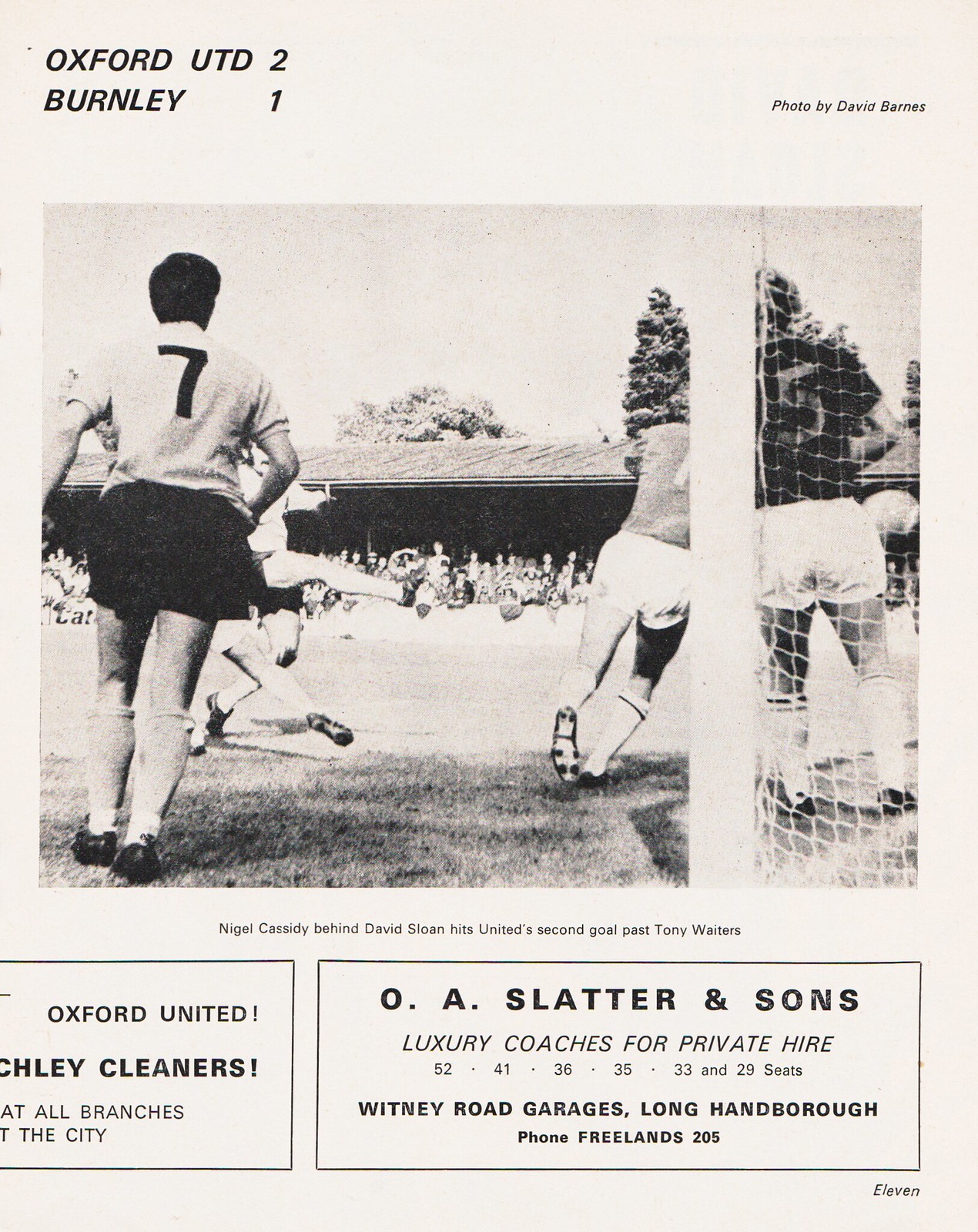This black and white poster, reminiscent of a vintage newspaper or old magazine page with an off-white background, measures approximately six inches tall and five inches wide. At the top left, bold black print announces "Oxford UTD 2" with a line below stating "Burnley 1." In the top right, “Photo by David Barnes” appears in small black letters. Dominating the page is a black and white photograph depicting a soccer match. 

On the right side of the image, a partially visible soccer net frames two players. The player nearest the edge, wearing white shorts, white socks, and a dark jersey with the number 5, stands slightly obscured by the net and the other player beside him, who sports a lighter-colored jersey. To the left, another player with brunette hair, dressed in a jersey with the number 7, dark shorts, and lighter socks, faces away from the camera. Behind him, the crowd is visible through an open space, partially sheltered. 

Below the photograph, in fine black print, the text reads, “Nigel Cassidy behind David Sloan hits United's second goal past Tony Waiters.” The bottom section of the poster features two rectangular advertisements. The left box, partially cut off, mentions "Oxford United cleaners at all branches..." The right box advertises "O.A. Slatter and Sons luxury coaches for private hire," listing seat capacities and contact details: “52, 41, 36, 35, 33, and 29 seats. Whitney Road Garages, Long Hanborough, Phone Freelance 205.”